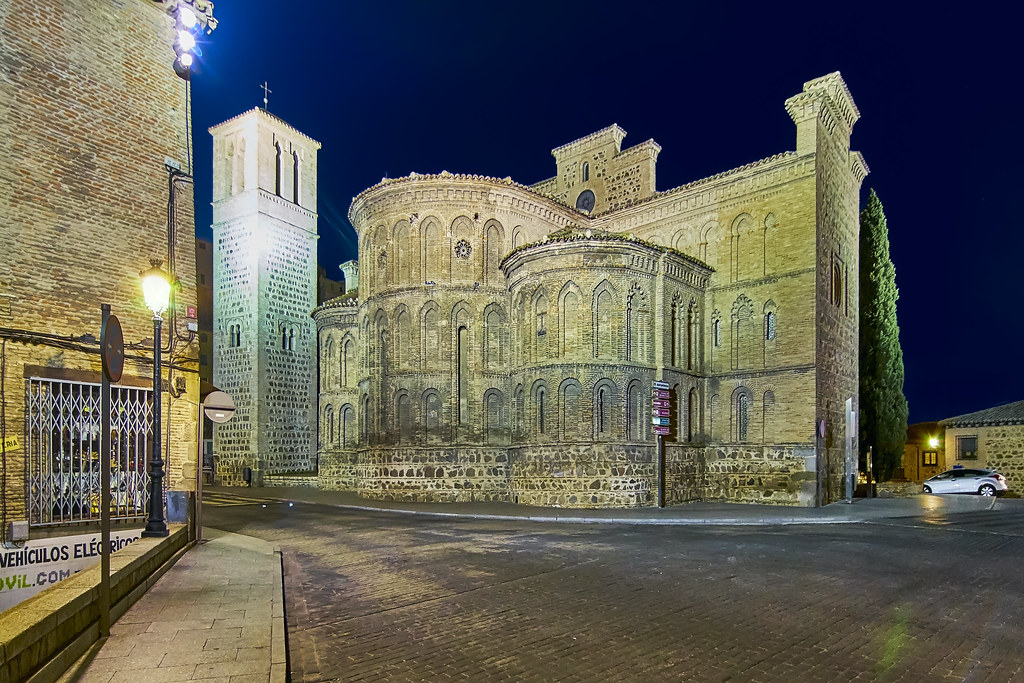This image, likely taken at night in a European city, features a historical setting capturing two prominent old buildings and various other urban elements. Dominating the scene is an all-brick building positioned centrally and slightly towards the left, resembling what might have once been a church. Its tall, arched windows have been sealed with additional brickwork. Adjacent to this, to the immediate left, stands a rectangular, three-story building with a possible lookout area on the middle level and a tall, skinny structure with a cross atop it, suggesting it is part of the church complex. A car is parked in the middle right of the frame, underscored by the gloom of the night and illuminated by streetlights emanating from the left. The street scene is dotted with street lamps, signage in an unrecognized language, and colorful elements including white, lime green, red, black, bright white, yellow, oxidized green, gray, and blue hues reflecting off the buildings. The setting gives off a tourist attraction vibe, where visitors might frequent for its historical and architectural significance.